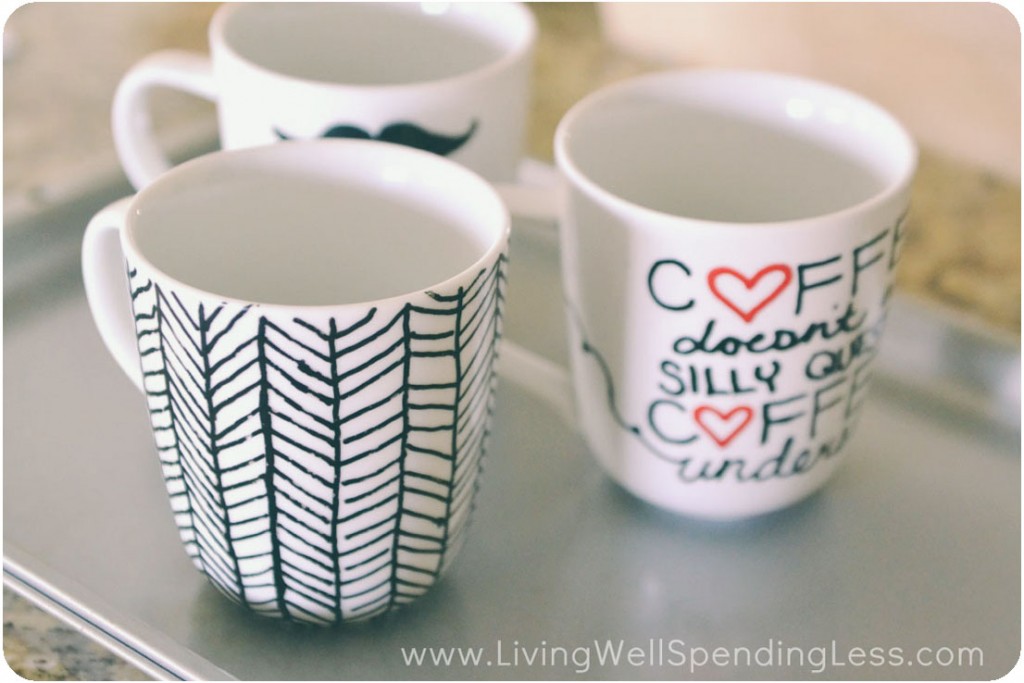The image features three white ceramic coffee cups arranged on a silver metal tray, likely placed on a granite countertop. The front cup sports a black and white design with intricate lines that resemble a leaf or web pattern. To its right, the second cup displays text where a red heart creatively replaces the 'O' in "coffee," and reads something along the lines of, "Coffee doesn’t understand," though the full text is not clearly visible. The third cup, partially hidden behind the first two, prominently features a mustache icon. At the bottom right, the image includes a website citation: www.livingwellspendingless.com.